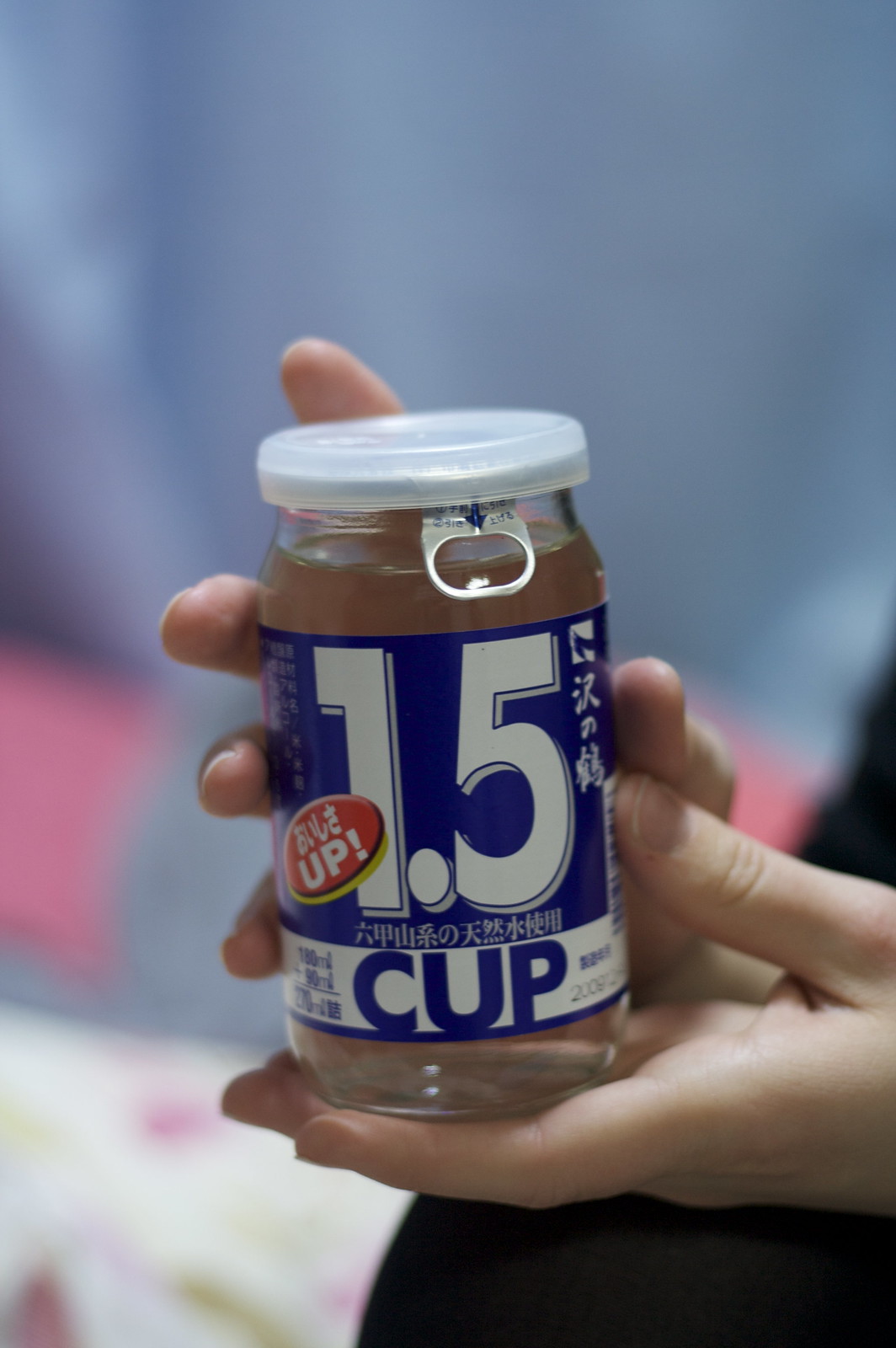In this vibrant, color photograph with a portrait orientation, a pair of human hands prominently features. One hand lays flat beneath a clear plastic container, while the other hand supports the container from above, fingers gently curved around its surface. The clear container, marked "1.5 cup" on its label, allows for the visibility of the hand cupping it from behind. A striking red circular label with the word "Up!" in bold exclamation point is affixed to the container. The container also has a white, metallic-looking lid equipped with a pull-tab, reminiscent of those found on drink cans.

In the background, figures or objects are barely discernible, blurred beyond recognition. Hues of blue dominate the out-of-focus backdrop, interspersed with touches of red, lending a dynamic yet subdued ambiance to the scene. The person holding the container is dressed in black, offering a stark contrast to the clear and colorful elements in their hands.